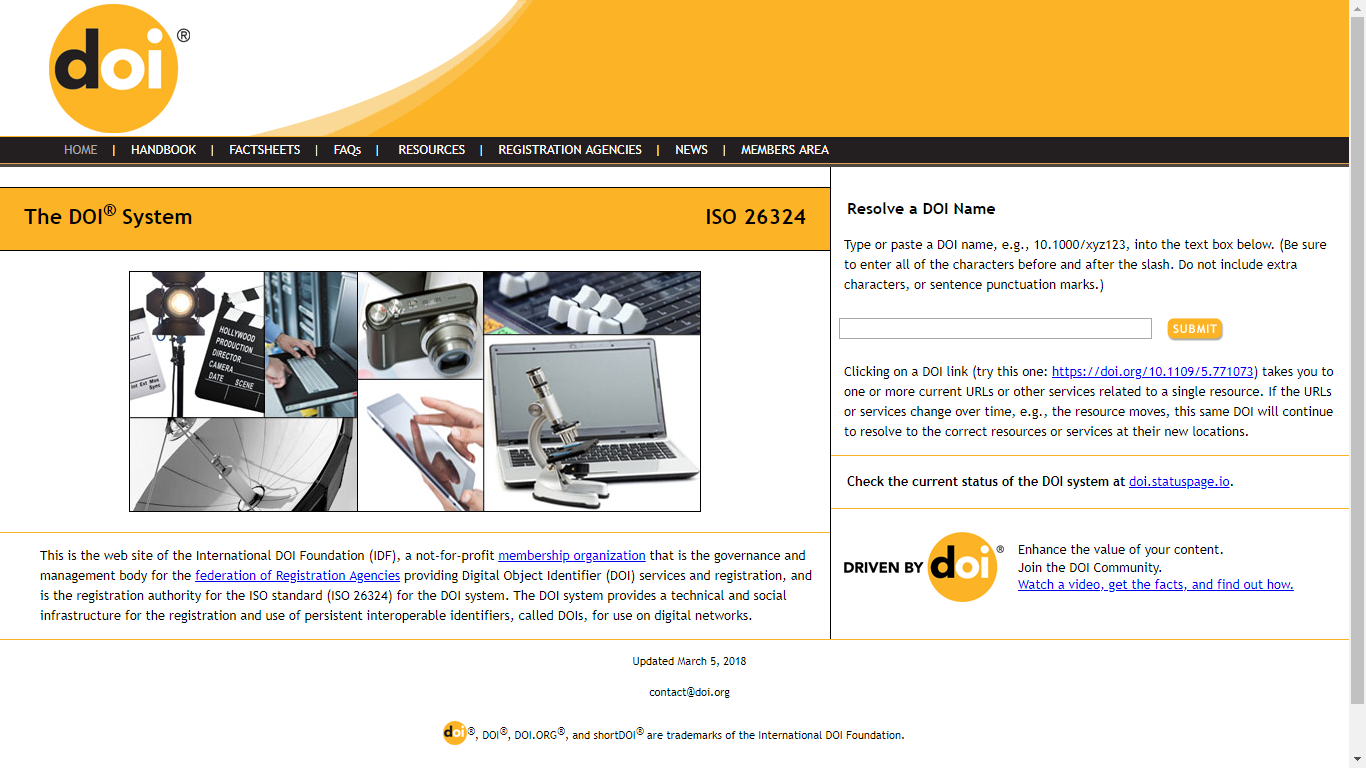A detailed description of the website depicted in the screenshot:

This image showcases a screenshot of a website dedicated to the DOI (Digital Object Identifier) System, prominently featuring the organization's visual identity. The DOI acronym is displayed, with the 'D' in bold black lettering, and 'OI' in contrasting yellow, all encapsulated within a solid yellow circle.

The website's top navigation bar is sleek and black, with white text for easy readability. The navigation options include: Home, Handbook, Fact Sheets, FAQ, Resources, Registration Agency, News, and Member Area. Beneath the navigation bar, there is a spacious white section followed by a yellow bar with a black border. Inside this bar, "The DOI System, ISO 26324" is inscribed in black letters.

The body of the webpage contains six images of various electronic devices and tools: a microscope, a computer keyboard, a phone, a tablet, a camera with lighting equipment, and a clapperboard, which are displayed in a horizontal row.

Further down, there is a section titled "Resolve a DOI Name," which provides a field where users can paste a DOI name for resolution. The page is interspersed with multiple paragraphs of explanatory text and descriptions, guiding users on the functionalities and utilities of the DOI System.